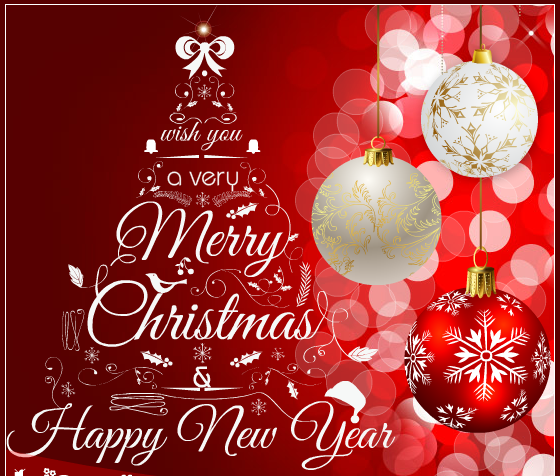This digitally created, Christmas-themed graphic features a detailed composition set against a maroon to red gradient background. The left side of the image showcases a Christmas tree made up of various decorative elements such as swirls, filigree, bells, leaves, and mistletoe, forming a triangular shape. Within this intricate tree design, text wishes viewers "a very Merry Christmas and Happy New Year," with the lettering increasing in size towards the bottom. Positioned at the tree's pinnacle is a white bow. The right side of the image displays three hanging Christmas ornaments: the top ornament is white adorned with gold snowflakes; the middle ornament is silver with gold filigree; and the bottom ornament is red with white snowflakes. The overall style suggests it might be intended for use as a festive e-card or part of a Christmas advertisement.